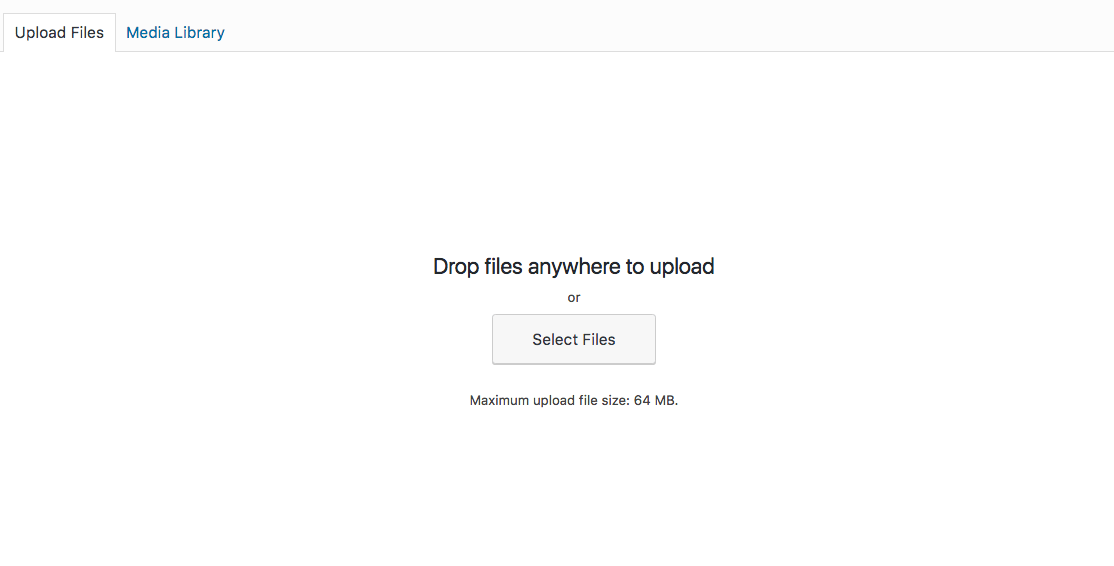The image displays a user interface for uploading files. The top section features a gray bar, with the words "Upload Files" in black text on the left. Adjacent to this, in blue, is the link "Media Library". Below this header, the background transitions to white. Dominating the center is a message stating, "Drop files anywhere to upload." Directly beneath this message is a rectangular gray button with the text "Select Files" centered within it. Lower still, a note indicates the "Maximum upload file size: 64 MB." There's a distinctive line resembling the edge of a folder tab running upwards and to the right, before turning back down near the "Upload Files" section, and then extending horizontally across the width of the interface. Beyond this demarcation, the background remains a continuous expanse of white.